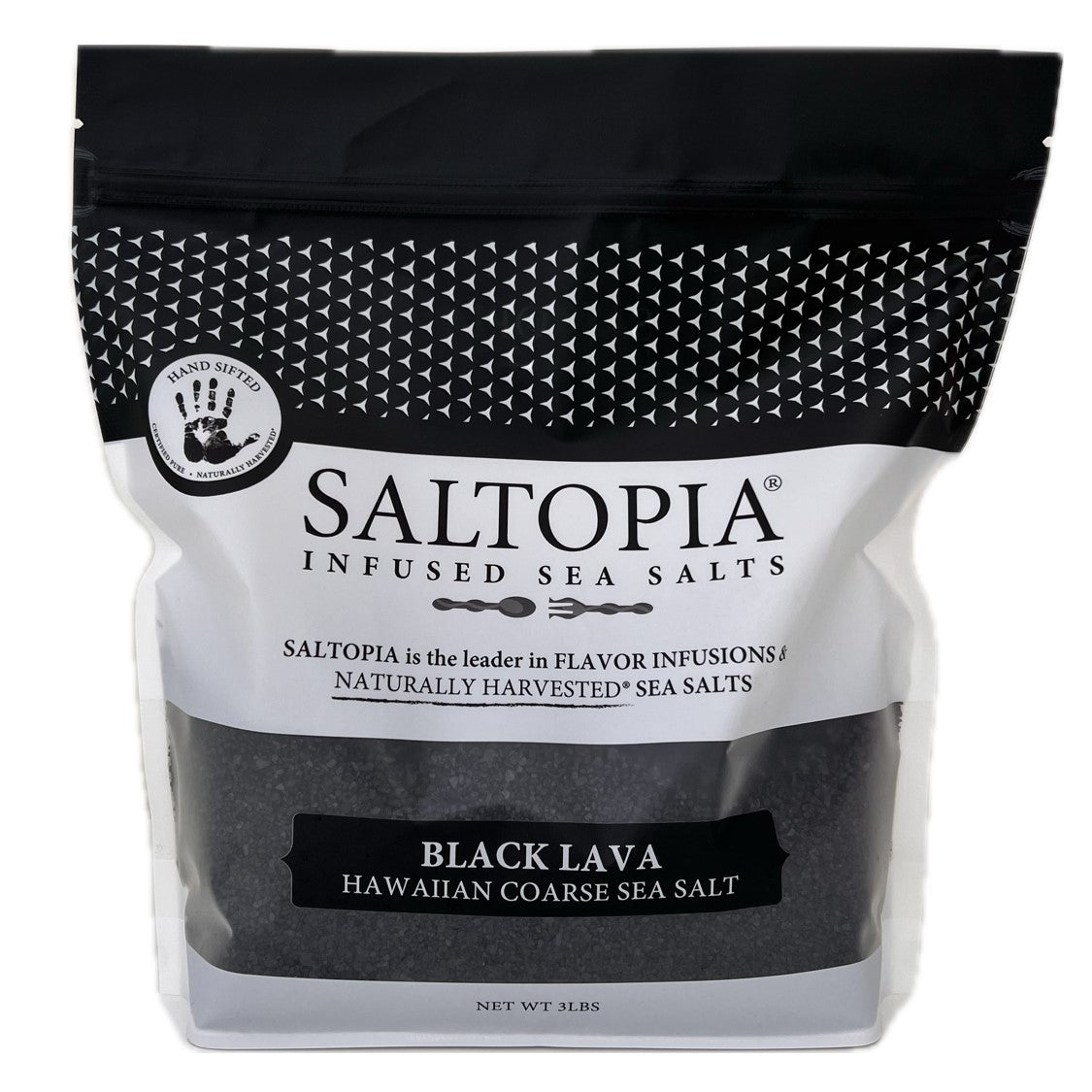This detailed image depicts a bag of Saltopia's Black Lava Hawaiian Coarse Sea Salt. The bag features a distinctive design with a black top adorned with a black and white pattern, followed by a central white strip that prominently reads "Saltopia infused sea salts" in black font. Below this central section, the bag showcases Saltopia's branding as the "leader in flavor infusions and naturally harvested sea salts," accompanied by a clip art image of a spoon and fork. A clear plastic window occupies the bottom third of the bag, providing a view of the black salt inside. The label within this transparent section reads "Black Lava Hawaiian Coarse Sea Salt" in white font on a black rectangle. Additional text on the top left corner highlights the qualities of the salt, stating "hand sifted, naturally harvested." At the very bottom of the bag, it designates the net weight as three pounds.